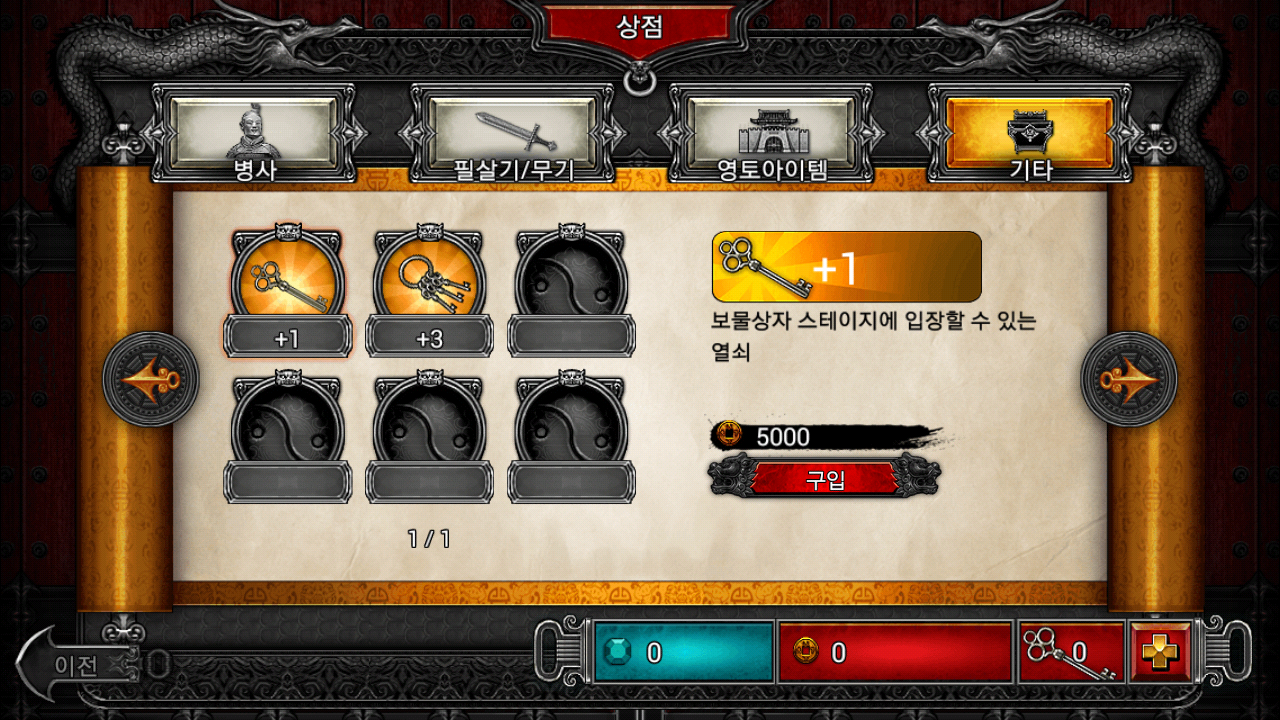The image is a color screenshot that resembles an online game interface, possibly from a computer game with an Oriental theme, dating back approximately twenty years. The dark black background contrasts with intricate elements and vibrant details. Grey dragon motifs frame the upper left and right corners, facing each other, adding an elaborate, mythical aesthetic. In the center, a large red rectangle with white Asian script is prominent, surrounded by a complex layout of smaller screens and objects.

To the right of the central red rectangle are two orangey-bronze pillars. At the top of these pillars are four small screens displaying a variety of symbols: a clown-like face, a sword, a robot, and a small black object, each accompanied by Chinese writing. Below these screens are six round grey objects, the first two illuminated in orange and yellow, with numbers one and three beneath them in white. An additional small circle sits to the left between the two rows.

Towards the right, an orange and yellow rectangle with a key symbol and a plus one is positioned, again accompanied by Chinese inscriptions. Below this, a smaller rectangle displays the number 5000 in Chinese writing. Another smaller red rectangle with Chinese text is beneath it.

On the far right side, a blue-to-red progress bar sits at the bottom, marked with numbers zero on both ends, and a key with zero on the right. A gold symbol adorns the far right end. The entire composition suggests a detailed and immersive gaming interface with elements indicating player status, score, and possibly health or progress metrics.